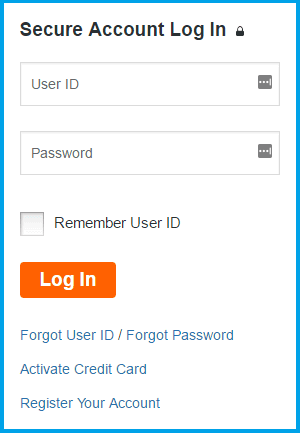The image depicts a secure account login interface. At the top, "Secure Account Login" is prominently displayed, accompanied by an icon of a lock, symbolizing security. Below this, there are two text boxes—the first labeled "User ID" and the second labeled "Password." Beneath these text boxes, there is an unchecked checkbox with the label "Remember User ID" beside it. Further down, an orange button with white text invites users to "Login." At the bottom of the interface, there is a collection of options written in blue text: "Forgot User ID/Forgot Password," "Activate Credit Card," and "Register Account." The entire image is succinct and focused on the elements necessary for user authentication.